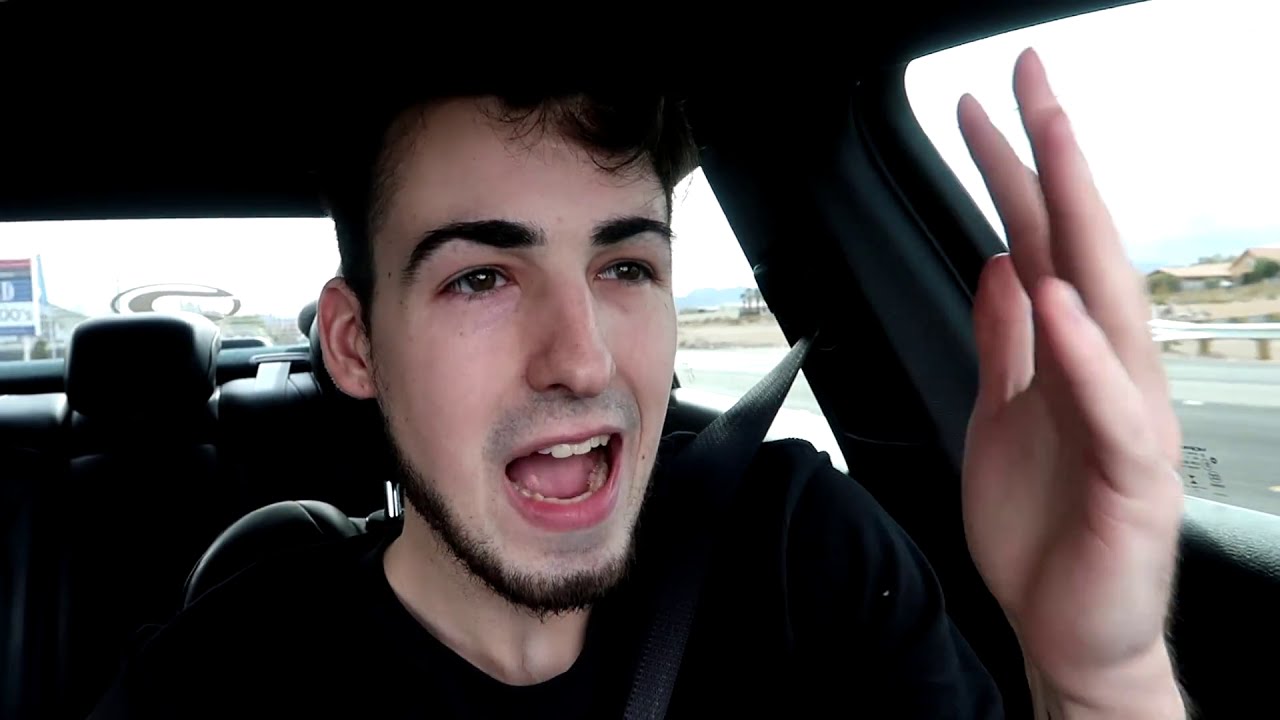The image depicts a young Caucasian man with dark hair, black eyebrows, and a short, neatly trimmed black beard in the driver's seat of a car, which appears to be a selfie possibly taken with a dash cam or his phone. The man is wearing a black T-shirt and his seat belt is visible across his shoulder and chest. His left hand is raised and pointing towards the 12 o'clock position. His mouth is open, giving the impression that he is talking or yelling, perhaps indicating a moment of road rage. The image captures the car's dimly lit interior, predominantly black in color, making it difficult to discern specific features. The exterior shows an overcast day with a gray road, a guard rail on the right, a hint of a street sign in the back window on the left, and the background includes a brown house with green bushes. His expression and posture suggest he is focused ahead, with his eyes directed towards the windshield.